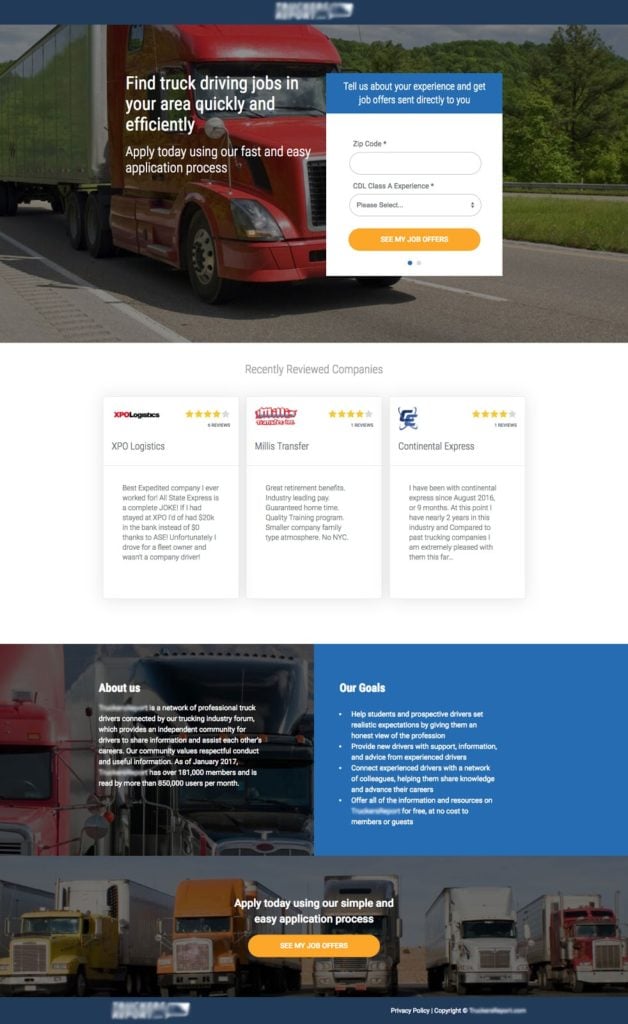The web page belongs to a trucking business, showcasing a promotional image to attract potential truck drivers. The main image features a vivid red semi-truck traveling towards the viewer on a busy freeway, with a silver-grey trailer in tow. Superimposed on the image is informative text that reads: "Find truck driving jobs in your area quickly and efficiently. Apply today using our fast and easy application process."

Additionally, a pop-up box on the image prompts visitors to provide details about their experience to receive tailored job offers. It includes fields for entering your zip code, and indicates if you hold a CDL Class A license, followed by a "See My Job Options" button.

Further down the page, there's a section titled "Recently Reviewed Companies," listing:
- XPO Logistics, rated 4 out of 5 stars
- Mills Transfer, rated 4 out of 5 stars
- Continental Express, rated 4 out of 5 stars

Unfortunately, the text of the reviews is too small to decipher. Toward the bottom of the page, there's an 'About Us' section which includes the company’s goals and reiterates their simple and efficient job application process. The page also features buttons encouraging users to "See My Jobs" and "Apply Today."